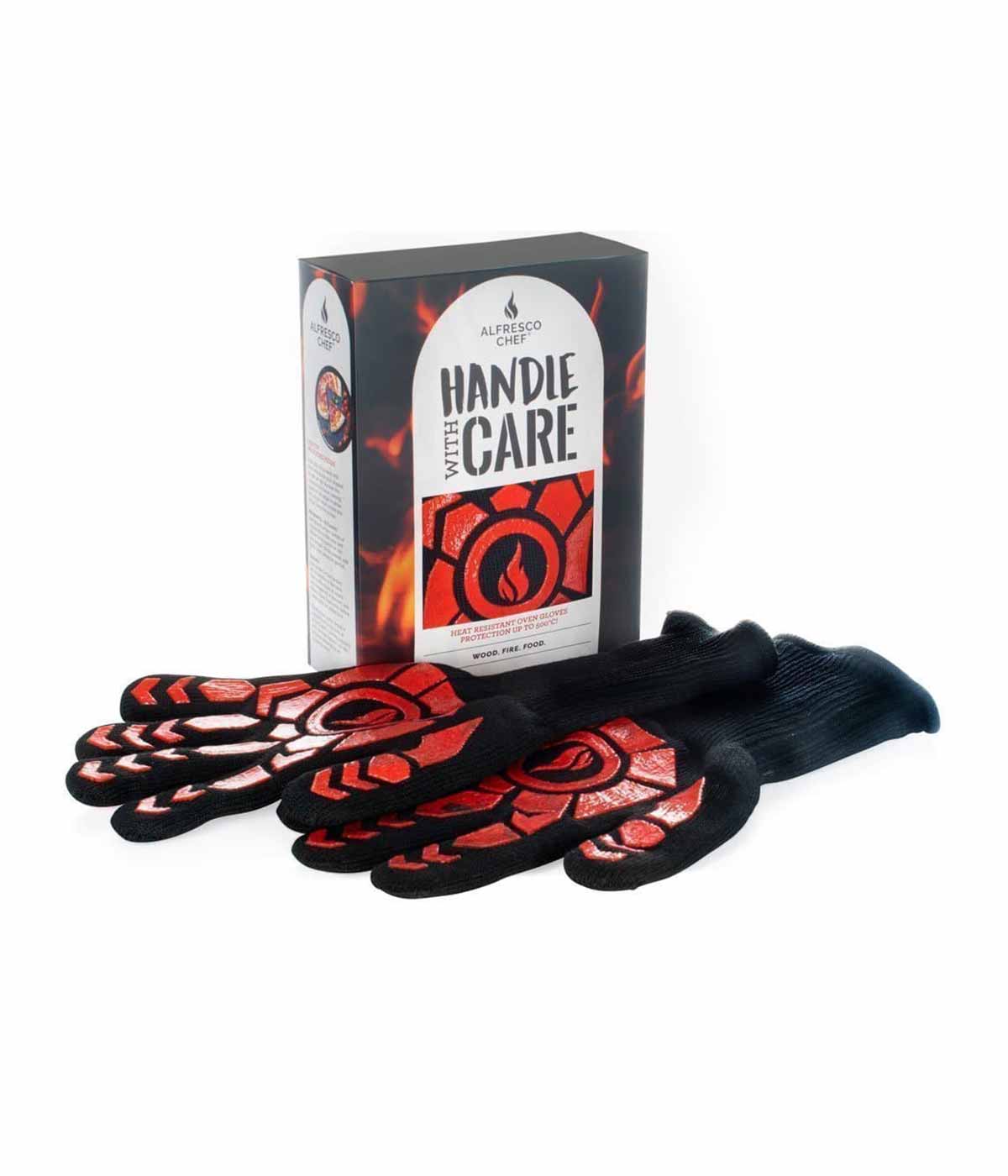This image showcases a pair of heat-resistant oven gloves specifically designed for culinary use, particularly for grilling or handling hot pots and pans. The gloves, branded as Alfresco Chef Handle with Care, are predominantly black with striking red accents on the fingers and palm, which feature patterns resembling arrows, hexagons, and circles. These red areas likely indicate a heat-resistant material to protect the user’s hands. A distinctive flame logo is positioned in the center of the glove's palm, reinforcing its heat-resistant capabilities.

The gloves are presented alongside their packaging, a sleek black box with white and red elements and a backdrop of flames, emphasizing the product's purpose. The box features a prominent "Handle with Care" label and an illustration detailing the glove’s inner sole, highlighting its red flame design. On the left side of the box, a white block with illegible text is visible. Set against a clean, white background, the overall presentation resembles a professional product mock-up typically seen on e-commerce websites.